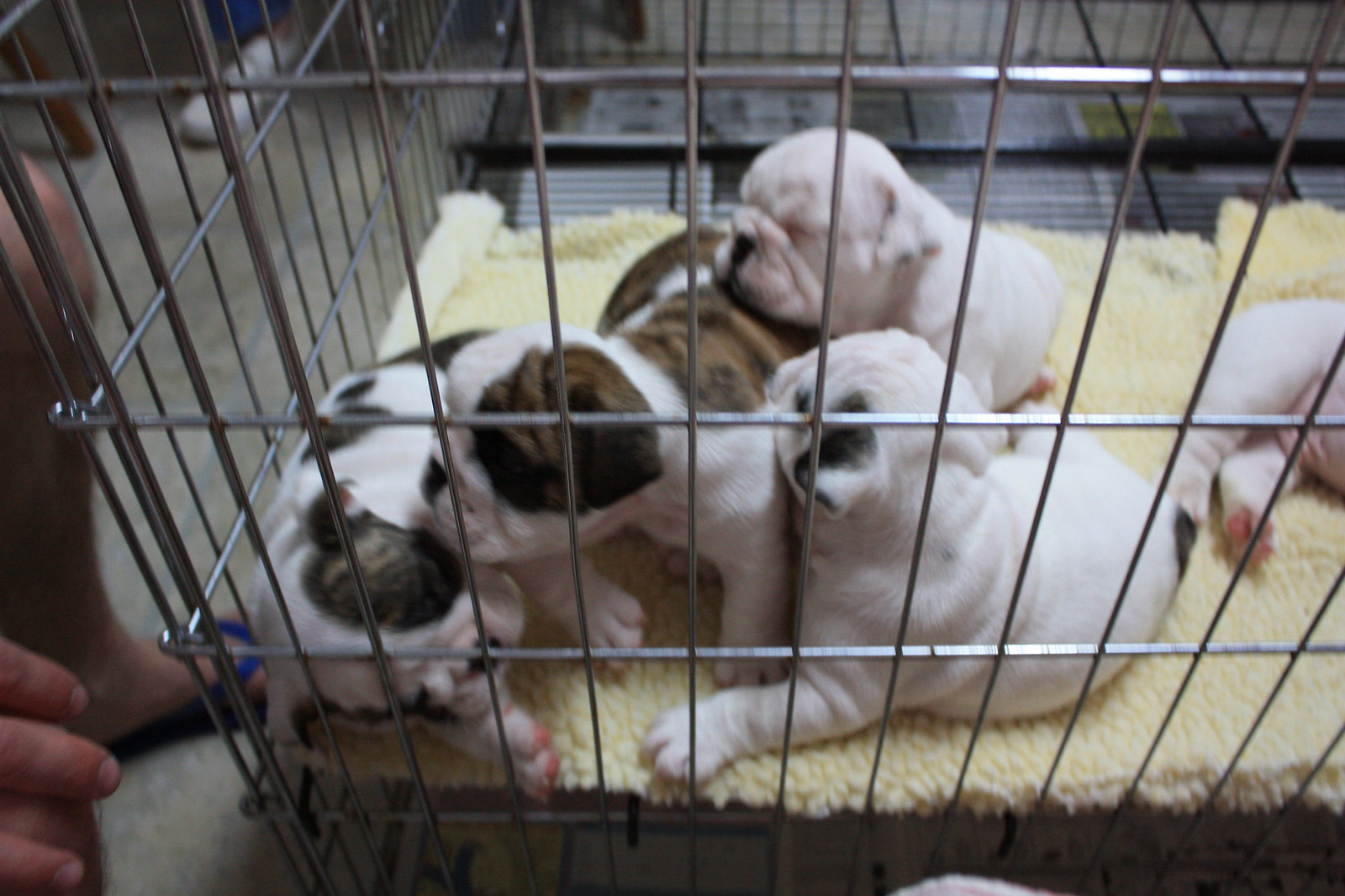This photograph captures six adorable bulldog puppies nestled together in a metal cage with a light yellow fleece lining. Their colors vary from predominantly white with small brown markings to a mix of brown and white, with some featuring distinctive brindle patterns. The puppies are sleeping peacefully, with one puppy adorably resting its head on another’s back, showcasing their pink paw pads and wrinkled noses. To the left side of the image, a person, semi-visible, is seen through their hand with short fingernails and their foot in a blue sandal. In the background, another cage and a person dressed in blue pants and white sneakers can be seen. The composition emphasizes the coziness and warmth of the puppies’ environment, made comfortable by the soft fleece underlay.